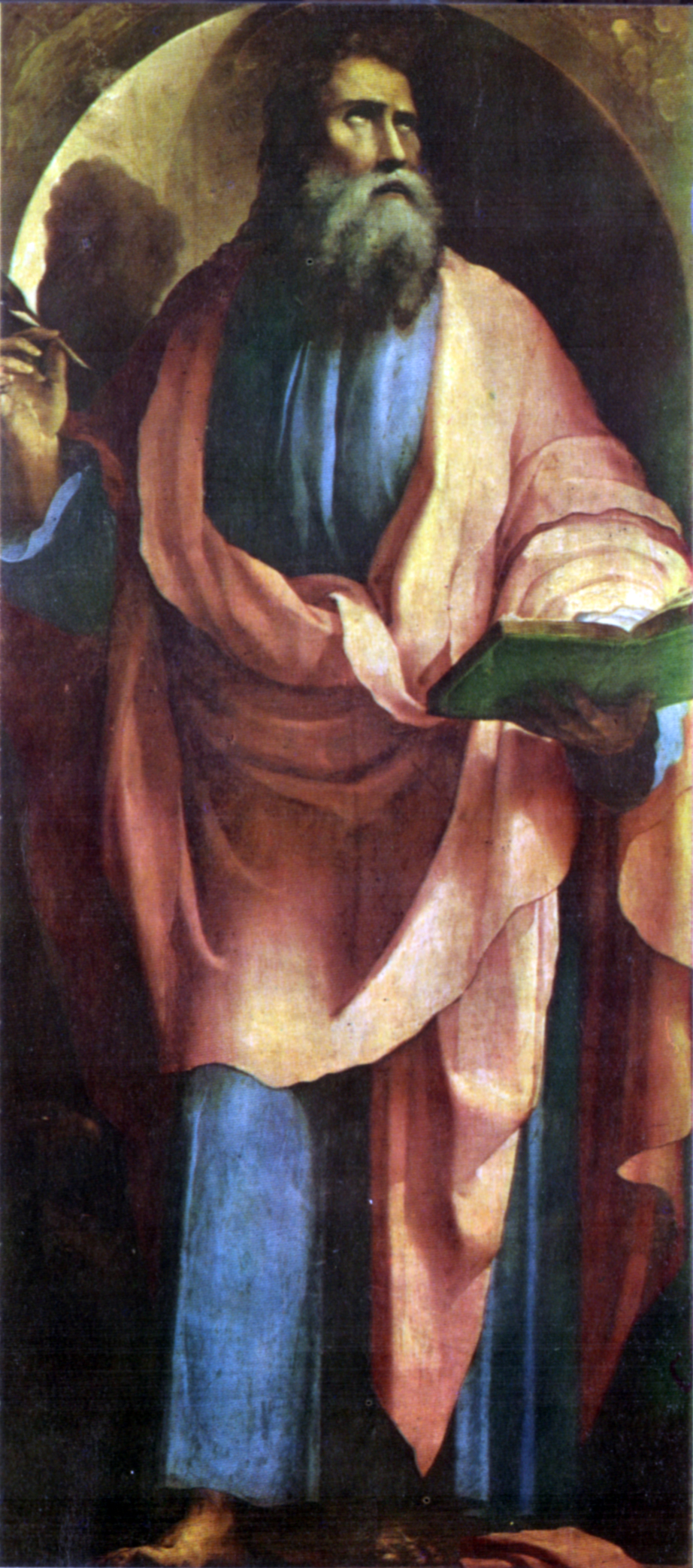This vertical rectangular painting features a man who occupies nearly the entire frame, from head to bare feet. He stands within an arched niche set in a stone wall, casting a shadow to his left. His complexion is medium, and he has long brown hair accompanied by a thick white and dark brown beard and mustache. He gazes upward to his right with eyes that appear almost entirely white, suggesting a visionary or introspective moment. His right arm is raised, bent at the elbow, holding what appears to be a paintbrush. His left hand holds an open green book at waist level, as if he had been reading before something captured his attention. The man is dressed in a blue shirt and pants, over which he wears a light beige or peach-colored robe that wraps around his shoulders and waist, flowing down to his legs with visible ripples in the fabric. The painting's darker lower section adds depth and contrast to the illuminated figure.